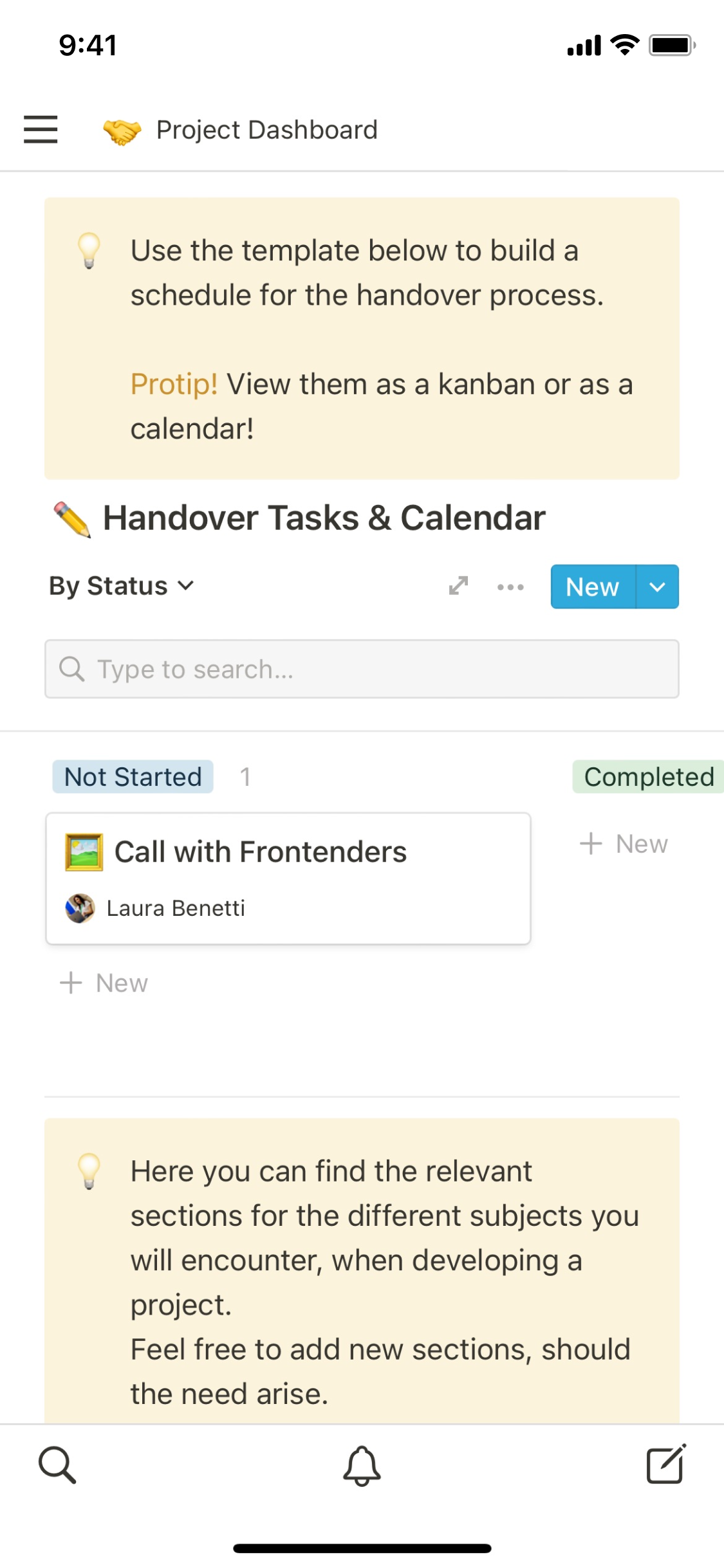At the top left of the image, the time is displayed beside the label "Simonet devices" which reads 9:41. In the top right corner, various icons are visible, including a signal bar labelled "Nesox," a Wi-Fi icon, and a battery indicator. Central to the image is a prominent header that reads "Project Dashboard."

Below this header, a template is outlined with instructions that guide the user on how to build a schedule for the handover process. A pro tip suggests viewing tasks as a Kanban board or a calendar. The tasks can be sorted by status, with one example provided as "Not started: Call with front-enders."

Further down, descriptive text explains the layout: "Here, you can find the relevant sections for the different subjects you will encounter when developing a project. Feel free to add new sections should the need arise." 

At the very bottom of the image, a notification bell icon is visible. To the bottom left, there is a magnifying glass icon representing a search function, accompanied by another notification icon.